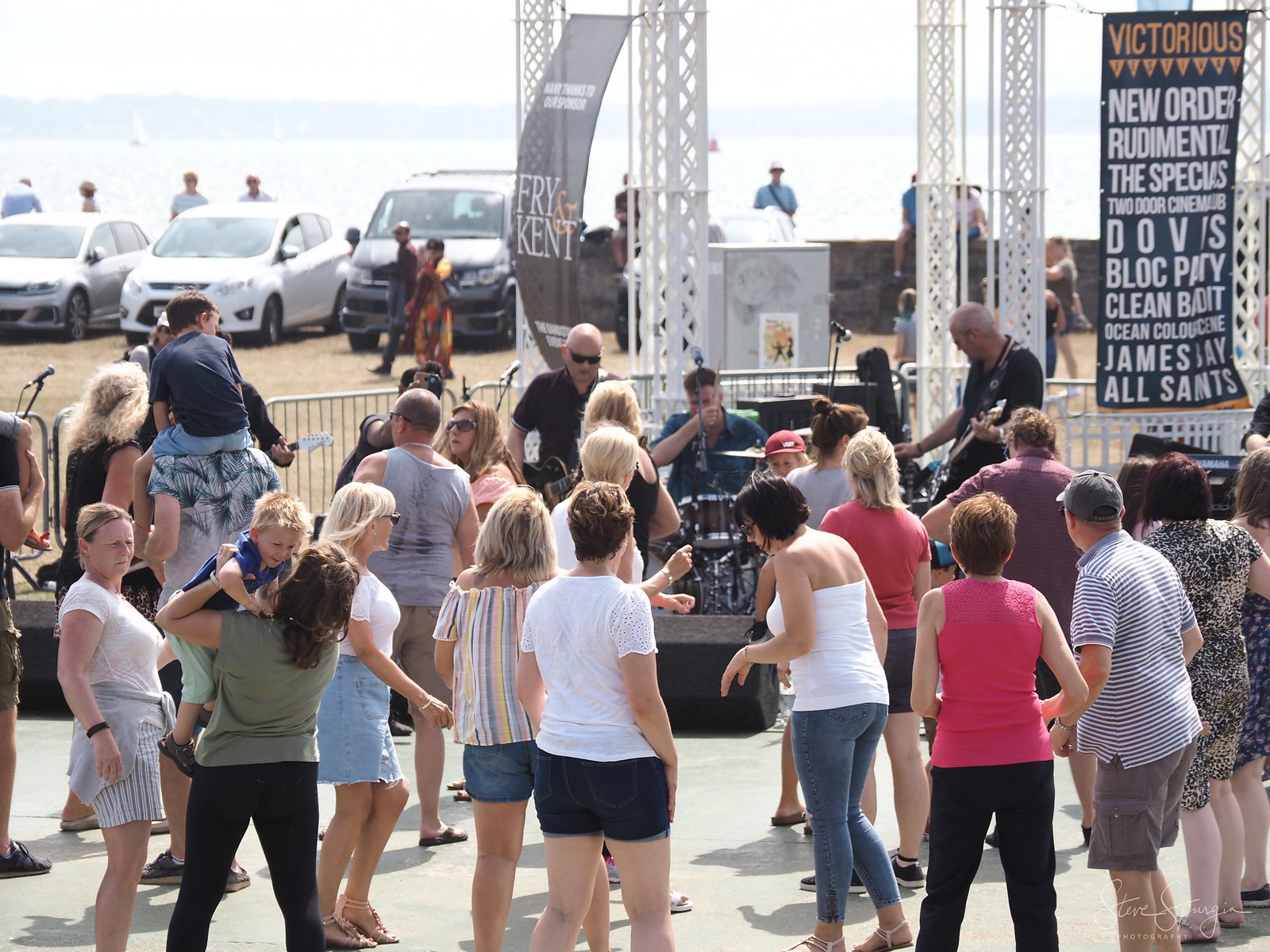In this vibrant image, we witness a lively outdoor music festival set against the picturesque backdrop of a beach. In the immediate foreground, a large crowd, many clad in shorts and short sleeves, suggests a warm, sunny day. They are gathered around a performing band, which includes two bald guitarists and a drummer wearing a hat. The band stands on a white stone-like ground, with metal fencing behind them signaling the boundary of the venue.

Dominating the top right of the image is a slightly wavy black banner hanging from white scaffolding poles. The banner prominently displays "Victorious" in orange text, followed by a list of bands in white text: New Order, Rudimental, The Specials, Two Door Cinema Club, Block Party, Clean Bandit, Ocean, James Bay, and All Saints. Parts of the banner are obscured due to folds, but its festive message is clear.

In the middle ground, parked cars and more festival-goers are visible, mingling on a light tan surface. Stretching beyond this bustling scene, we see a sandy beach with people standing and enjoying the day. The expansive body of water glistens under the sun, with distant mountains and sailboats punctuating the far horizon, enhancing the idyllic setting.